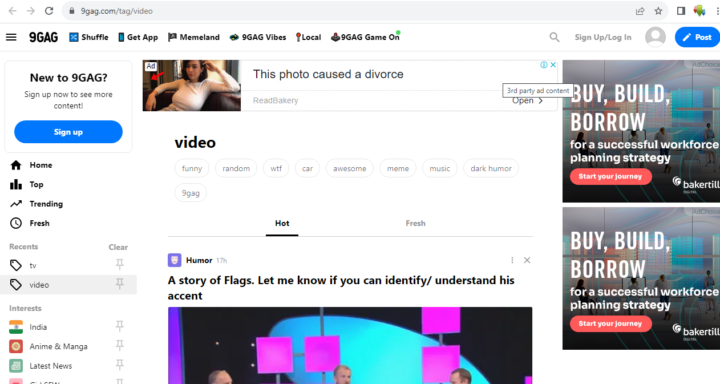This image is a cropped screenshot of the 9GAG desktop webpage. In the top-left corner, the 9GAG logo is prominently displayed. To its right, there is a horizontal navigation bar listing categories: "Shuffle," "Get App," "Meme Land," "GAG Videos," "Local," and "9GAG Game On." On the far-right end of this bar, icons and options include a magnifying glass for search, a "Sign Up" or "Log In" button, a blank profile photo placeholder, and a blue circle labeled "Post."

On the far-left side of the page, there is a vertical panel. At the top, it welcomes new users with "New to 9GAG?" followed by an encouragement to "Sign up now to see more content," and a blue "Sign Up" button beneath this message. Below this section, categories such as "Home," "Top," "Trending," and "Fresh" are listed vertically. Further down in this panel, "Recent" appears on the left with "Clear" to its right, followed by various tags.

Centrally located at the top of the page is an advertisement that reads, "This photo caused a divorce," with a clickable "X" in the far-right corner to close the ad. Directly below this, the label "video" is displayed in lowercase black bold print, accompanied by a selection of tags below it. Lower on the page, the sections "Hot" and "Fresh" are mentioned, with "Hot" being selected and showing content categorized under "Humor," followed by a specific story.

On the far-right side of the page, there are two identical ads for the "Workplace Planning Strategy Company."

This detailed description encapsulates the layout and key elements present in the screenshot of the 9GAG webpage.